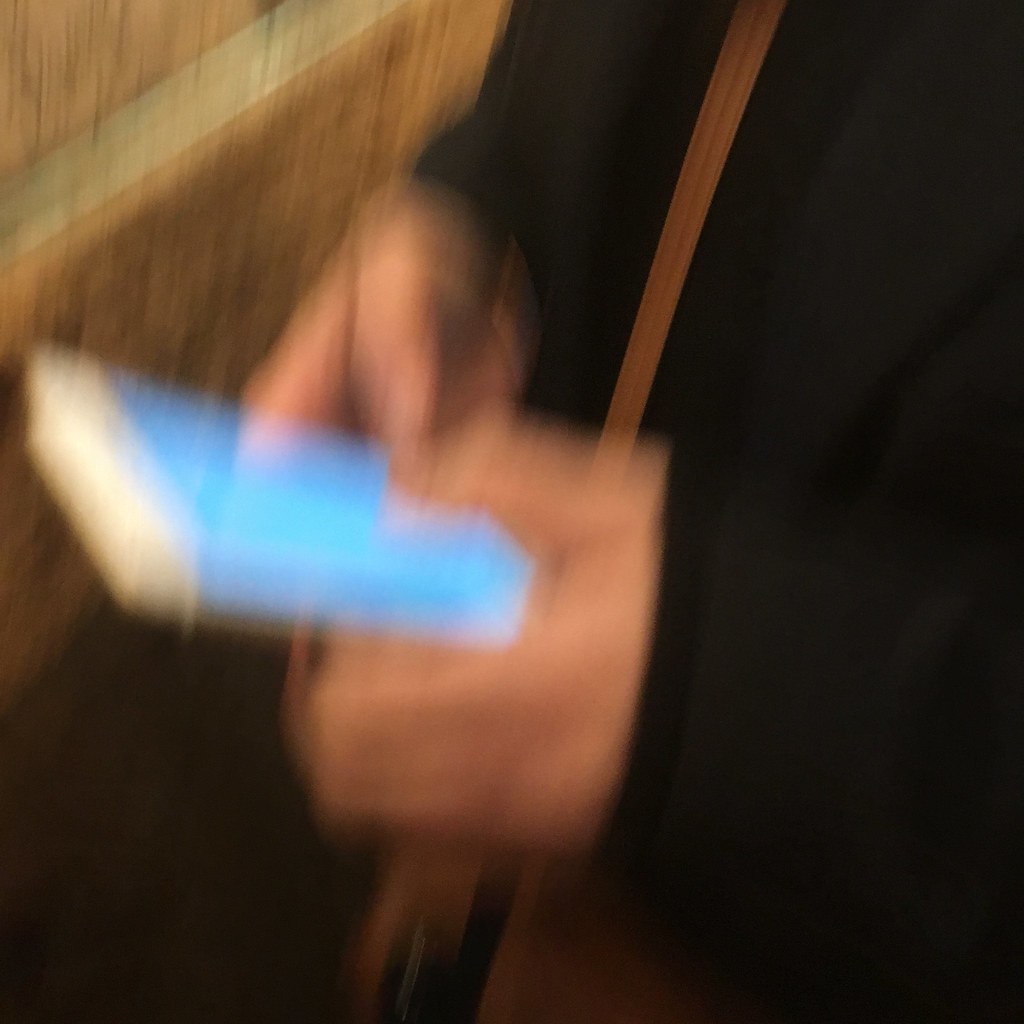A highly blurred photograph captures an individual holding a digital smartphone with both hands, actively typing on it. Due to the blur, the content on the phone's screen is indiscernible. The person is wearing a black coat or jacket and has a side bag adorned with a light brown strap. They are positioned in front of a brick wall featuring a mix of brown and light grey bricks held together by cement, with water stains visible in some areas. The blurriness of the image obscures many finer details, and there is a noticeable lack of color differentiation and saturation, suggesting that the picture was likely taken accidentally or hastily, perhaps by someone seated nearby.